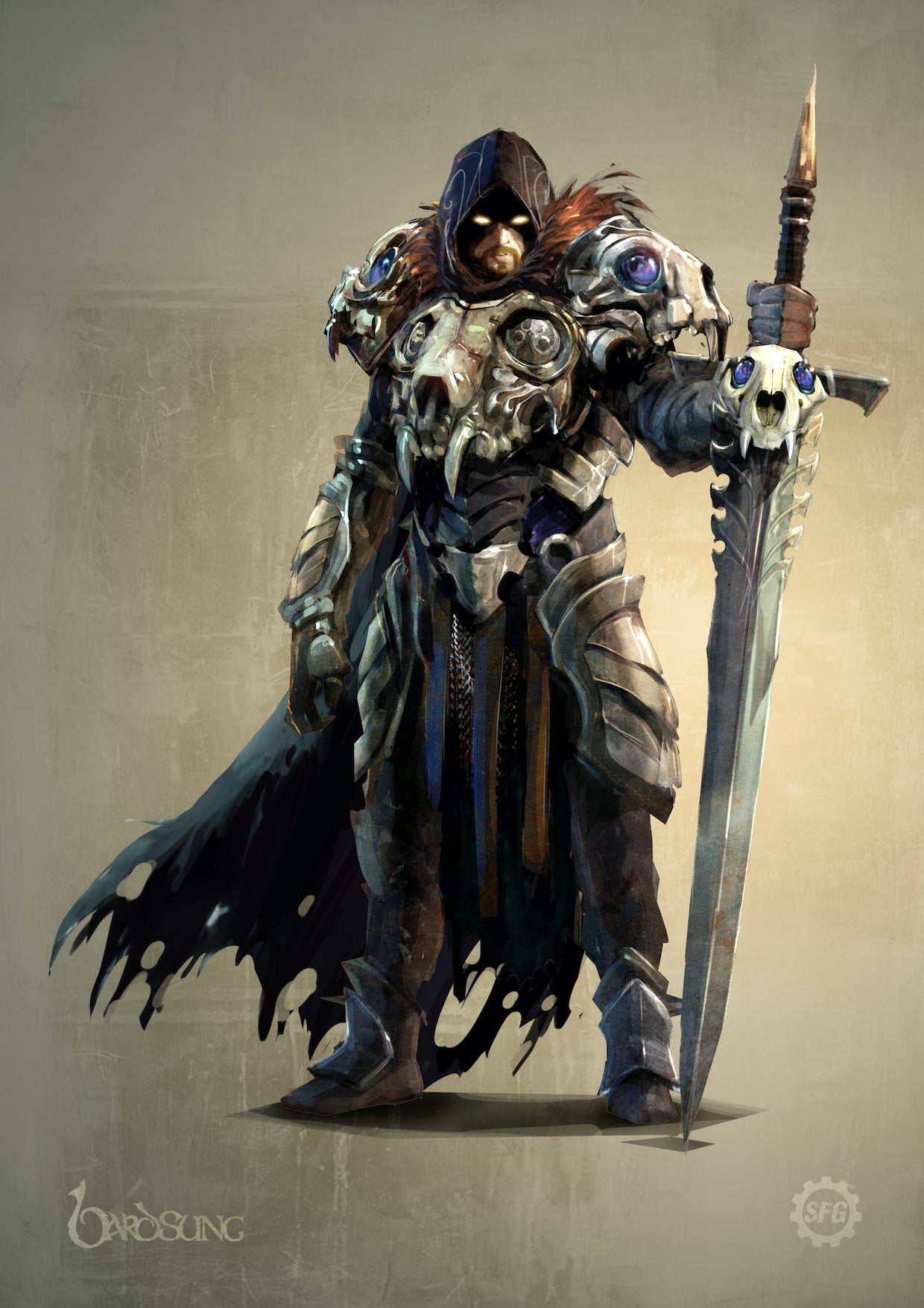In this highly detailed digital artwork, we see an imposing warrior character, seemingly from a role-playing video game. The composition is vertically rectangular with a background blended in shades of gray and light brown, devoid of definitive scenery. Notable details include watermarks: “Baro Sung” in a distinctive, non-cursive font on the bottom left, and a white or light tan gear icon with the letters "SFG" in the center, positioned at the bottom right.

The character himself is encased in heavy, protective armor that appears both formidable and intricate. His gear includes metal guards on his shoulders, thighs, feet, and particularly the chest and genital areas. Distinctively, the shoulder and chest armor are designed to resemble the skull of a creature, featuring large eyes, nostrils, and two prominent sharp teeth, which add a menacing touch to his appearance.

The warrior sports a tattered, hole-filled cape that flows behind him, and he wears a cowl over his head, revealing yellow eyes and a goatee. In his left hand, he grips a massive greatsword, which is stabbed into the ground. This sword is taller than the character himself, with a hilt adorned with another creature's skull similar to those on his armor. The blade’s handle extends above his head, suggesting that even its base could be used as a weapon. The blade is serrated near the hilt and sharp at both ends, enhancing the weapon's lethal design.